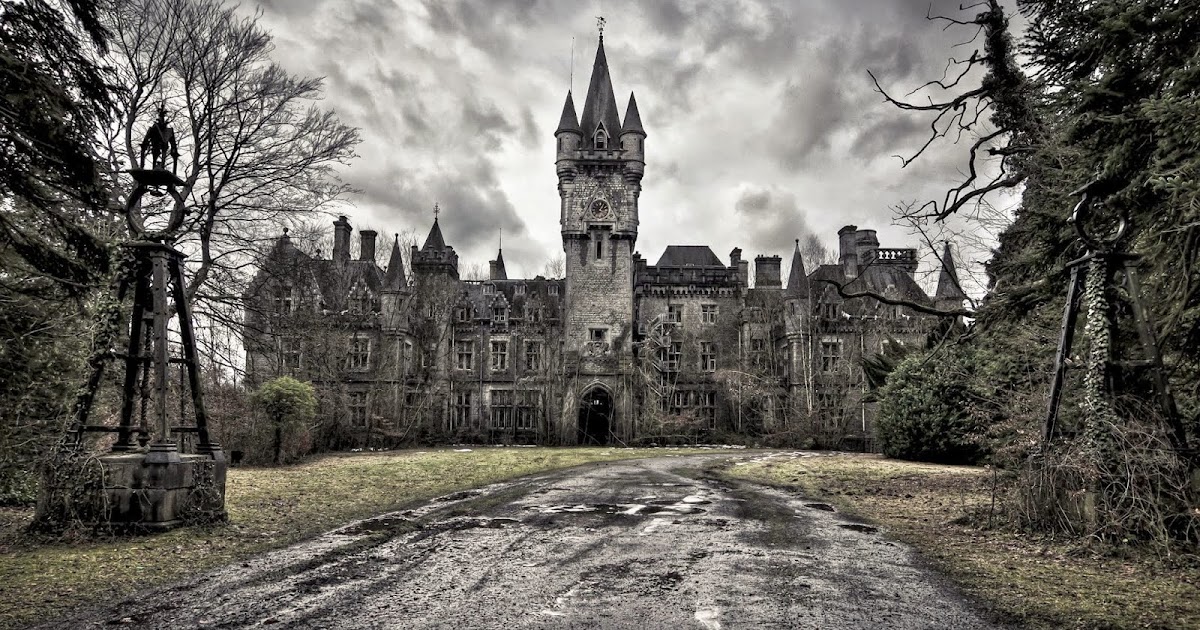The photograph captures an imposing, abandoned castle set against a backdrop of a very cloudy, gray sky. The image has a predominantly black and white tone, with only a hint of green from the grass visible in the scene. The castle itself is very large and features a central tower with turrets and spires, giving it an imposing height. Flanking the central tower are three-story sections, also adorned with smaller spires. The entire structure appears dilapidated and overgrown with vines, suggesting it has been neglected for a long time.

In front of the entrance, which is marked by a very large arched door, a gravel roadway leads up to the castle. On either side of this unpaved road are two unique lampposts, featuring a stone base and a steel pyramid structure topped with a circular design and lights. To the right at the top of the castle, there is a balcony, and several windows are scattered across the façade. Off to the side, there is a notable statue of a man. Tall, old trees surround the area, adding to the sense of abandonment and decay. The overall atmosphere is one of eerie desolation, emphasized by the overcast sky and lack of vibrant colors.